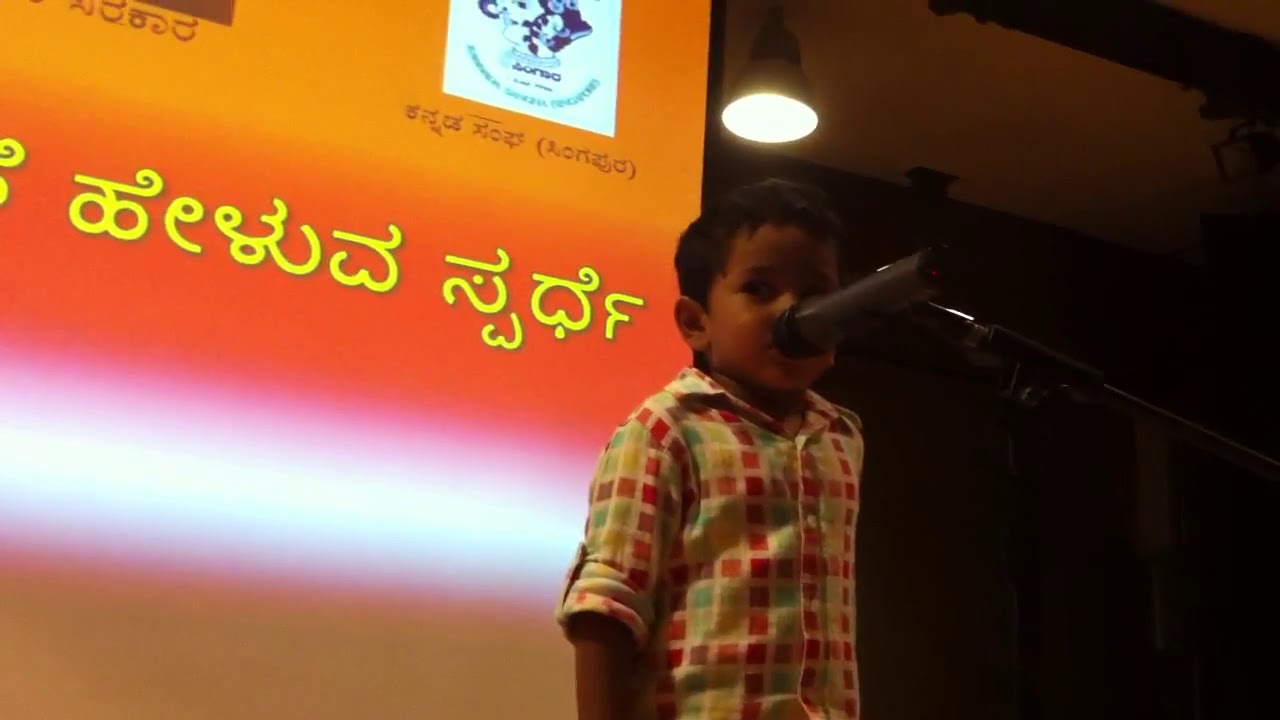In this image, a young boy with light brown skin and black hair stands at the center, singing into a microphone attached to a black stand. His mouth is pressed against the black microphone, which has a gray cylinder body. The boy is looking to the left, wearing a colorful plaid button-down shirt with rolled-up sleeves, featuring shades of red, light green, blue, orange, and yellow.

The setting appears to be an indoor space, possibly a gym or staged area, distinguished by a shaded ceiling light and a bright round lamp directly above the boy's head. The right side of the image is darker, indicating a stage or room extension. Behind the boy to the left is a tall display screen cut off at the top, showing a gradient background of yellow, orange, white, and brown bars. The screen includes an icon in a white square and cursive text in a foreign language written in brown and yellow colors, suggesting the image might have been taken in another country. The boy has a nervous expression, potentially indicating he's participating in a public speaking event like a spelling bee.